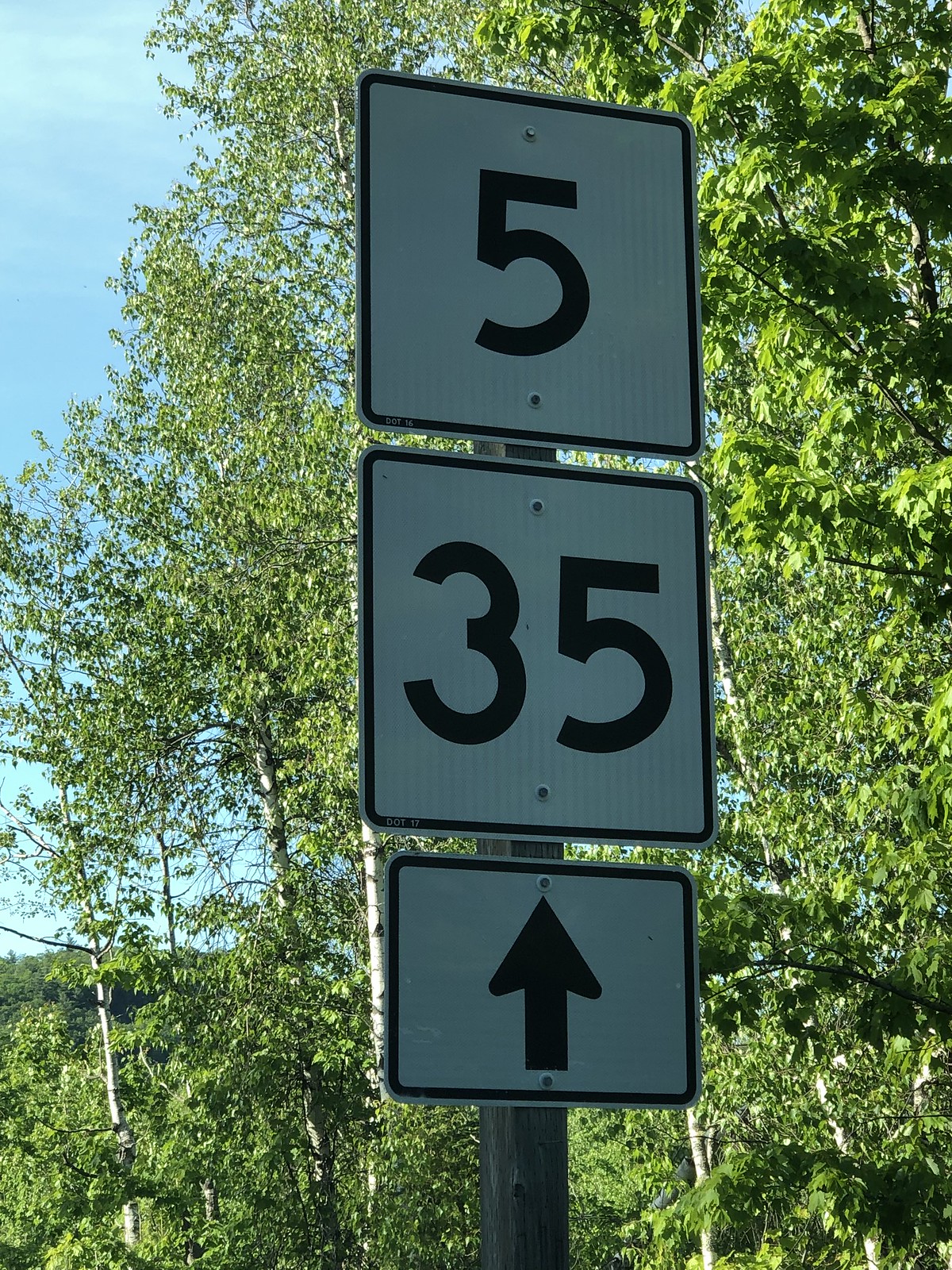The image captures a vibrant daytime scene, with a clear blue sky adorned by small, red-tinged clouds in the top left corner. The bright sunlight bathes the entire area. The majority of the background is dominated by lush, green trees. Centered in the image stands a black pole with three signs affixed to it. The signs, primarily white with black borders, are neatly arranged. The top sign is a square displaying the number '5' in black. Below it, another square sign shows the number '35' in black. The bottom sign, rectangular in shape, features a solid black arrow pointing upwards, indicating directions to highways or interstates '5' and '35'.